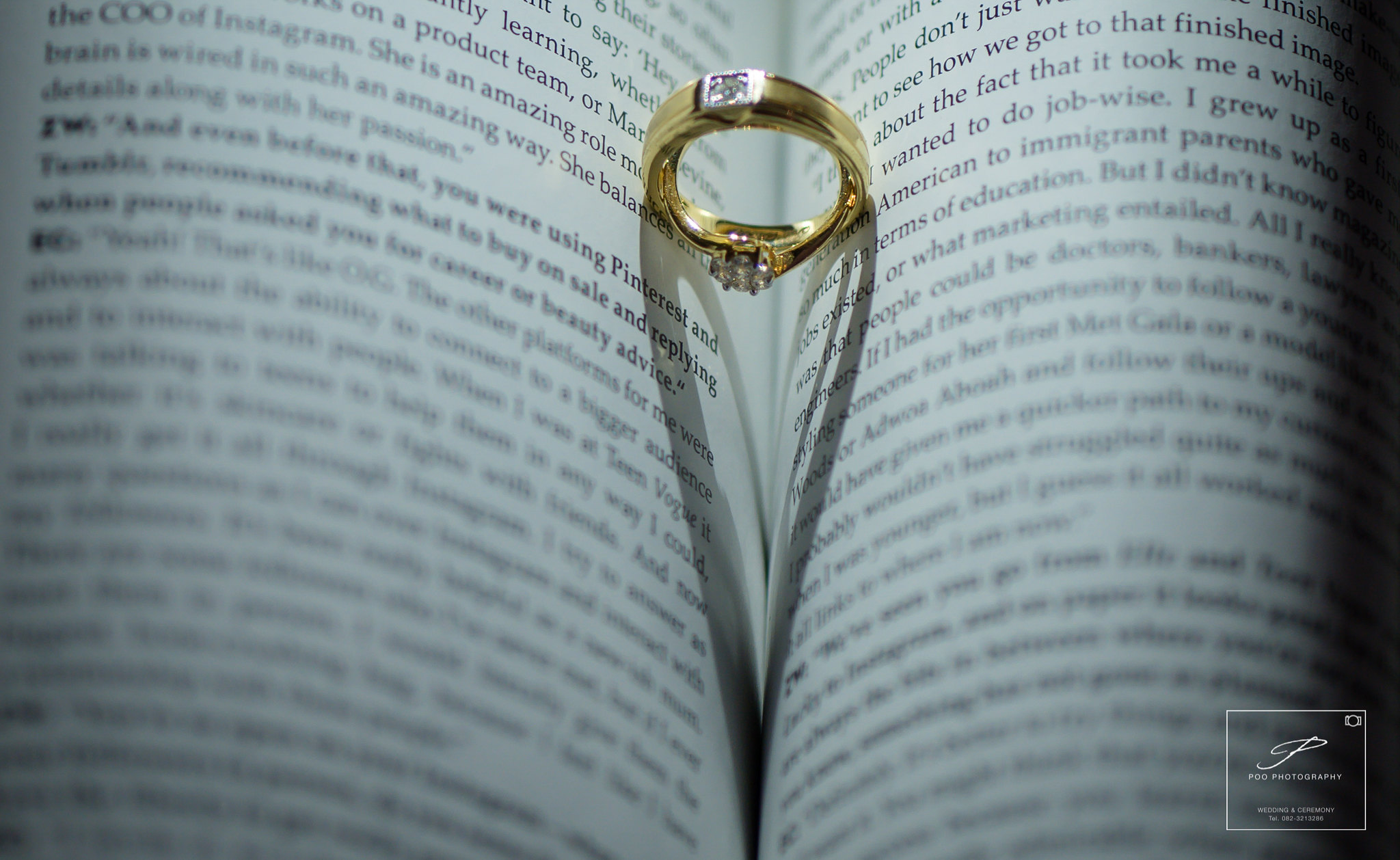The image showcases an open book or magazine with its pages elegantly curled on both sides, creating a rolling effect that frames the center crease. Suspended in the middle of this crease is a gold diamond ring, prominently featuring a square diamond at the top and another inset diamond at the bottom, which would actually be on the top when worn. The ring casts a heart-shaped shadow along the inner spine of the book, adding to the romantic aesthetic of the image. The print on the pages is largely illegible, with only snippets like “she is an amazing role model” and phrases that hint at career aspirations and an American context discernible. The background features a subtle bluish hue. In the lower right corner, there is a logo composed of a stylized letter "P" encircled in white, likely indicating the brand or photographer, with accompanying text that is too small to read.